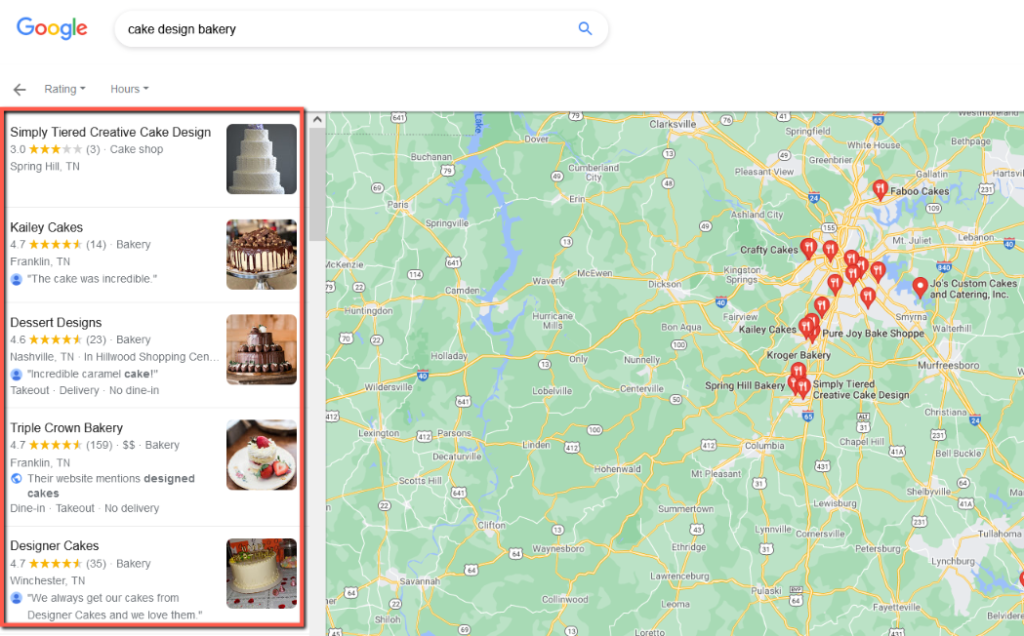This image showcases a Google search result page for "cake design bakery." In the upper left-hand corner, the recognizable "Google" logo is displayed. To the right of the logo is the search bar where the query "cake design bakery" has been entered.

Directly beneath the search bar, you can see a section that includes ratings and operating hours for the bakeries, accompanied by drop-down arrows for more details. Further down, there is a vertical menu listing different bakeries. There are five bakery listings in total: 

1. Simply Tie-Tiered Creative Cake Design
2. Kaylee Cakes
3. Desert Dessert Designs

On the right side of the page, there is a map pinpointing the locations of these businesses, giving a visual representation of where each bakery is situated.